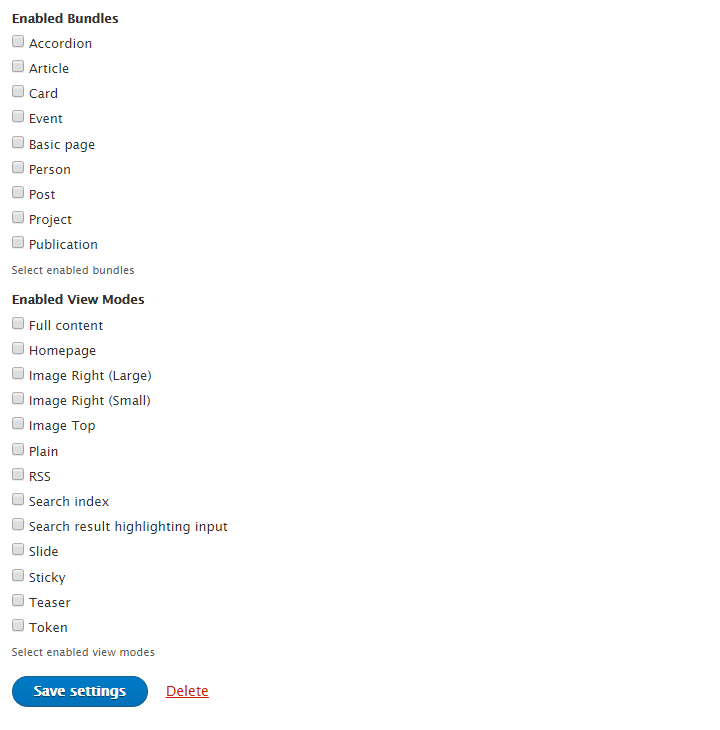This image is a vertical portrait screen capture, most likely from a web page, with a white background that merges seamlessly with the screen, making the image's boundaries indistinguishable. The central content is a list of items with clickable boxes on the left side, presented in black text on a white background. The entire layout is left-justified.

The image is divided into two main sections. 

At the top left, in bold black font, is the header "Enabled Bundles." Below this header are nine items, listed alphabetically:
1. Accordion
2. Article
3. Basic Page (with a lowercase "p")
4. Card
5. Event
6. Person
7. Post
8. Project
9. Publication

Each item has a gray square checkbox on the left, none of which are checked. Below this list, in smaller, left-justified font, the text reads "Select enabled bundles."

A small space below this, the second section begins with a bold header, "Enabled View Modes," with "E," "V," and "M" capitalized. This section lists thirteen items, again each with a square checkbox on the left, and none are checked. The items are listed in alphabetical order:
1. Full Content
2. Home Page
3. Image Right (Large)
4. Image Right (Small)
5. Image Top
6. Plain
7. RSS (all caps)
8. Search Index (with "index" in lowercase)
9. Search Result Highlighting Input (with only the "S" in "Search" capitalized)
10. Slide
11. Sticky
12. Teaser
13. Token

Below this list, in smaller font, the text reads "Select enabled view modes."

At the bottom of the image, aligned to the left, is a blue rectangular button with rounded corners and white text that reads "Save settings." To the right of this button is an orange-red text link, "Delete," which is underlined.

The overall image features a clean, left-justified design with a focus on functionality and clarity in presenting selectable options for web settings.